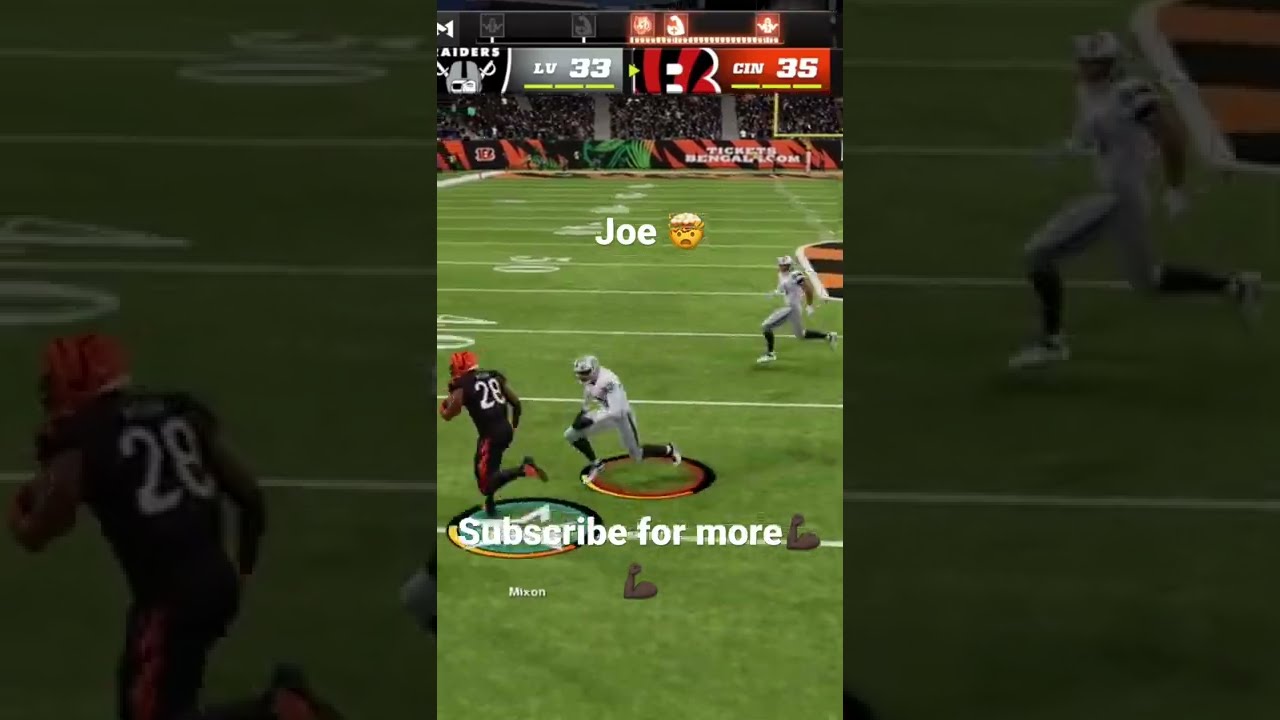This vertical image, likely a screenshot from a video game such as Madden, portrays a tense moment on an American football field. The scene is centered on a Cincinnati Bengals player, identified as number 28, Joe Mixon, clutching the ball and sprinting towards the left. He is donned in a black and white uniform with a red helmet, being pursued closely by a Las Vegas Raiders player in a silver and black uniform. Approximately ten yards behind, another Raiders player is also in motion, rushing to join the defensive play around the 38-yard line. 

In the background, the stadium is packed with spectators, reinforcing the intensity of the game. A partially visible field logo indicates this is taking place inside Cincinnati’s stadium. At the top of the image, the score is displayed prominently: Raiders (LV) 33 with their helmet logo and Bengals (CIN) 35 with their corresponding logo, each accompanied by three yellow bars. 

In the center of the field, the name “Joe” appears with an open-mouth emoji and, at the 30-yard line near his feet, the text "subscribe for more" is written in white letters. Beneath this text, an icon of a brown arm flexing its bicep is visible, adding a dynamic visual element. The left and right edges of the image are darkened, framing the vibrant action in the middle. This detailed visual encapsulates a thrilling snapshot of the game, urging viewers to subscribe for more exciting content.